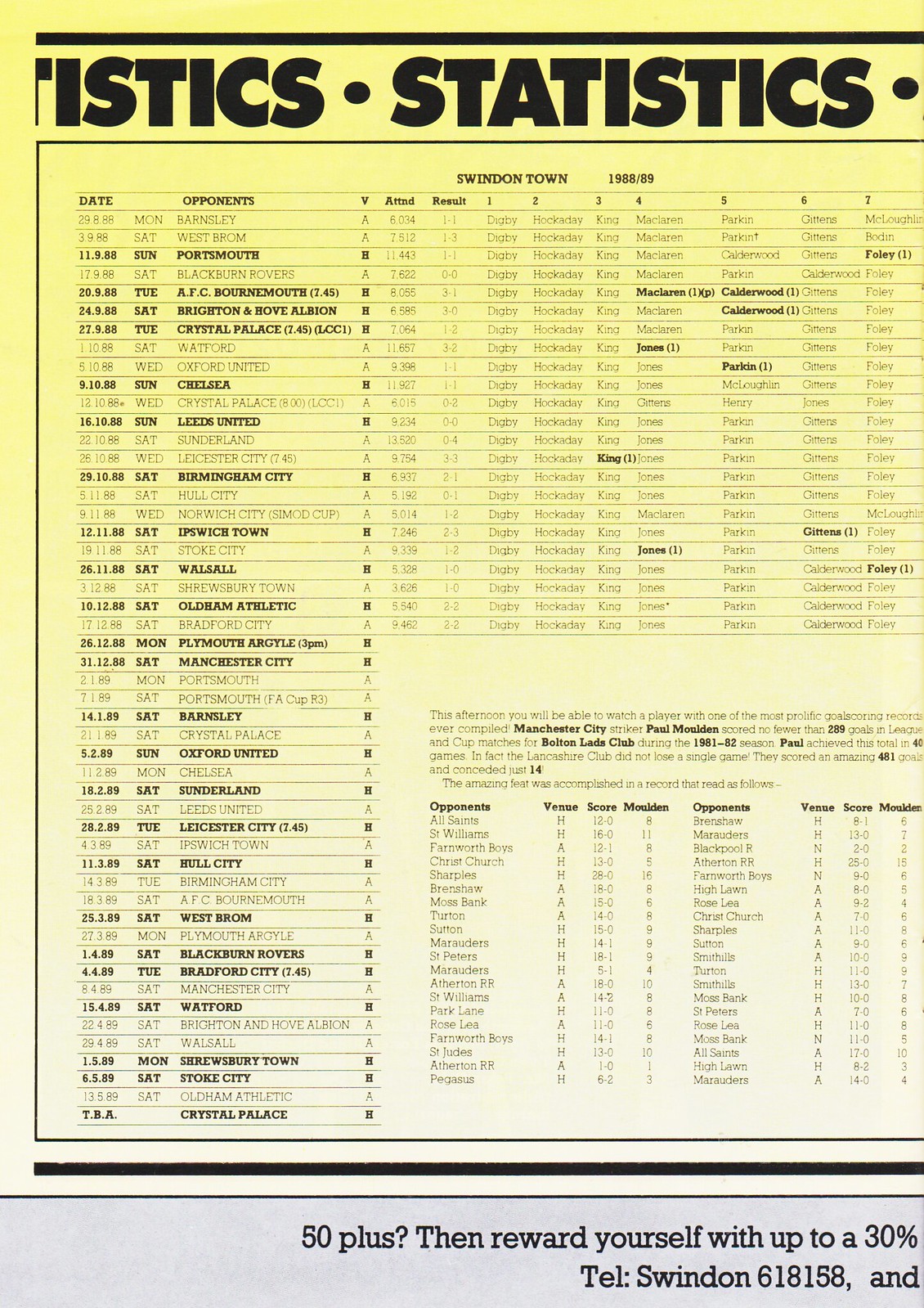The image depicts a close-up section of a page from a soccer statistics publication, possibly a book, magazine, or newsletter, focused on Swindon Town's 1988-89 season. The page starts with a bold black title "Statistics" on a yellow background that fades to white towards the bottom. The table organizes various data into rows and columns, with prominent headings including "Date," "Opponents," "V," "ATTND," and "Result." 

The first record shows the date "29.08.88," a Monday, with the opponent listed as "Barnsley," an 8 under "V," and an attendance figure of "6034." The result is noted as "1, 2, 1." Along the left-hand side is a list of dates and opponents, corresponding with recorded stats stretching across the page. The bottom of the table features a gray bar with a partial promotional message reading, "50 plus? Then reward yourself with up to a 30%," followed by a truncated telephone number "Sweden 618.158."